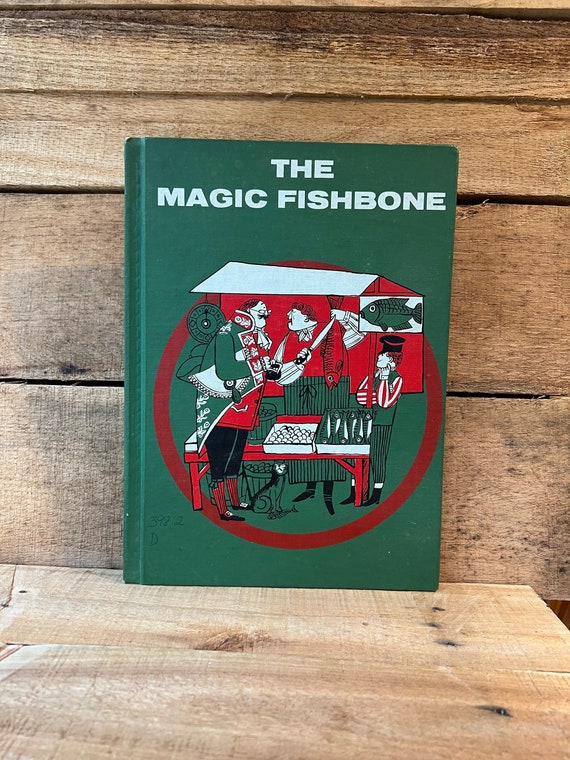The image is a vertically aligned rectangular photograph, likely taken indoors. It captures a medium brown, horizontal wood-planked wall that occupies the top two-thirds of the image. At the bottom is a wooden surface, possibly a bench, table, or countertop, which stops abruptly on the right side where a solid black area is visible.

Leaning against the wood wall is a hardcover book, primarily dark green in color. The book’s title, "The Magic Fishbone," is prominently displayed at the top in large, all-caps white print. Below the title is a striking red circle containing animated illustrations of three characters. The main scene shows two men conversing: one man in a large green jacket with white decorative elements, and another in a white shirt holding a knife next to a red fish on a table. A third, shorter man is also present near the setup, which includes various boxes, eggs, and another fish. The detailed, cartoonish artwork gives a whimsical feel to the book cover.